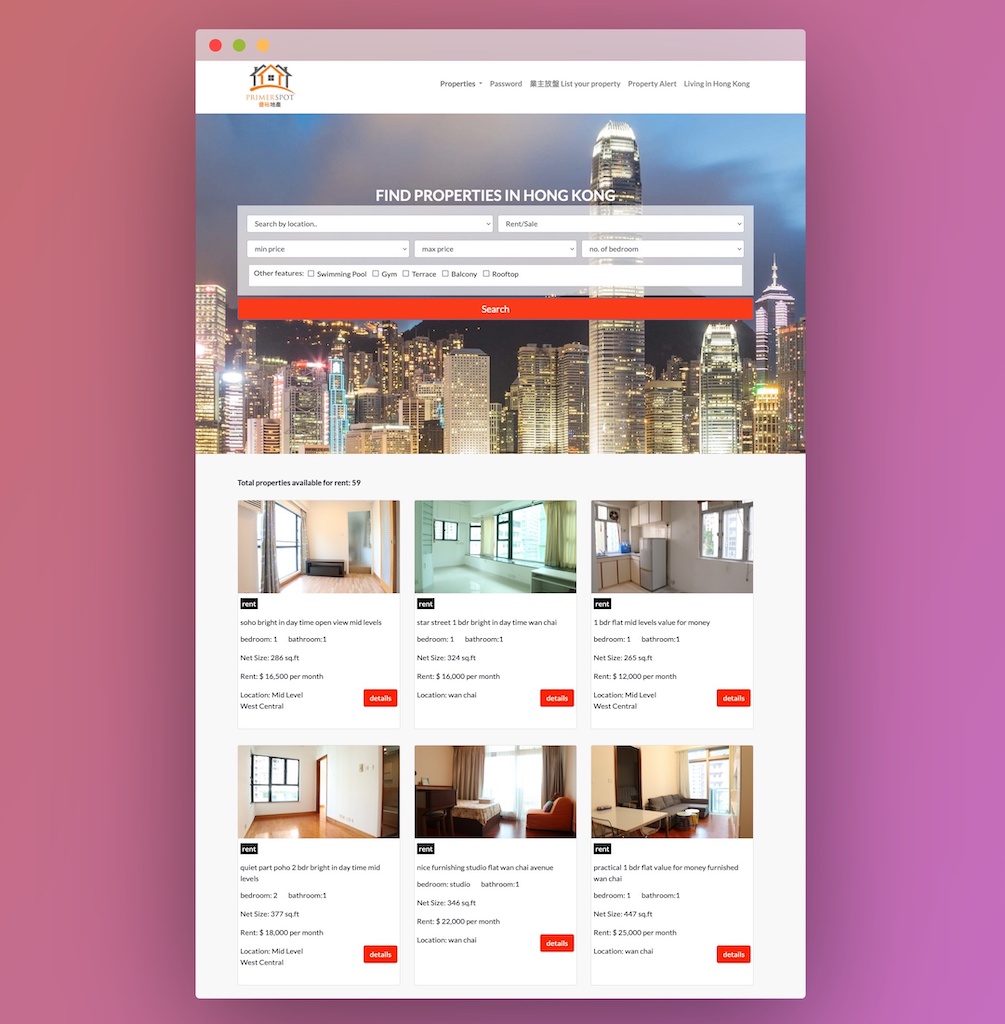This screenshot showcases a refined real estate search interface focused on properties in Hong Kong. The background is a soothing blend of purple and lavender hues. Dominating the screen are six prominent images, each depicting various luxurious hotel rooms, presented in a carousel or grid format that allows users to explore different options. The cityscape features the captivating night lights of Hong Kong, adding a vibrant urban touch. At the top, there is a search bar where users can type in specific addresses, and with a single click on the bold red search button, which is accented with white text and a distinctive emblem, the platform displays all available properties.